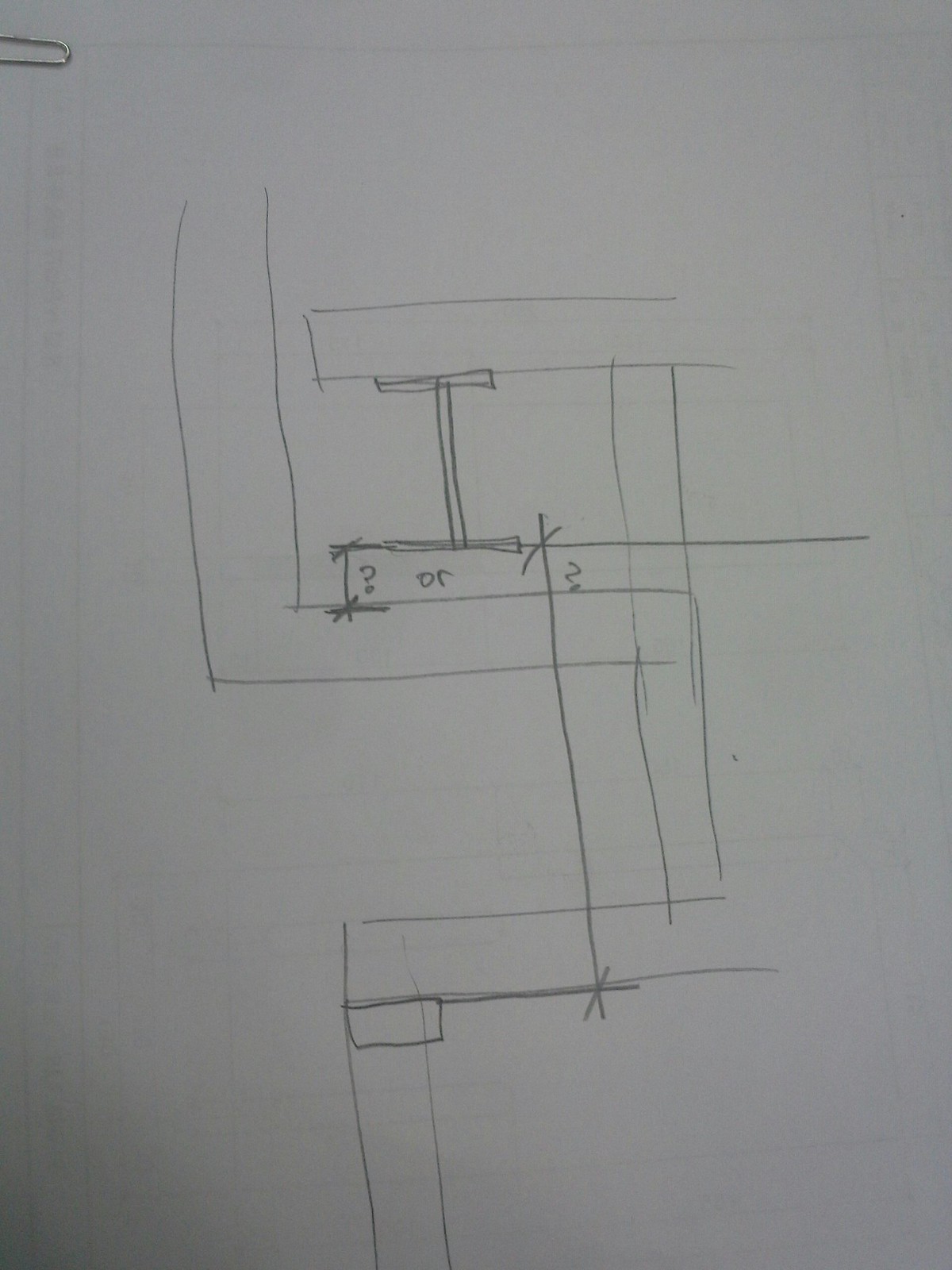The image features a photograph of a white sheet of paper displaying a highly intricate diagram, possibly a map. The primary element is a bold, dark rectangle that extends vertically downward and then bends at a sharp 90-degree angle to the right, forming an L shape. It continues in this horizontal direction before making another 90-degree turn downward for a shorter distance. Following this, the path takes yet another 90-degree turn to the left.

Above this L-shaped path, there is a complex T-shaped figure, which appears to support or intersect with another T-shaped form. These shapes are somewhat convoluted and difficult to describe accurately. Within the diagram, there is a question mark accompanied by the word "OR" inscribed nearby. The diagram's purpose and meaning are not immediately clear from the image alone, leaving the viewer puzzled about its exact intent or function.